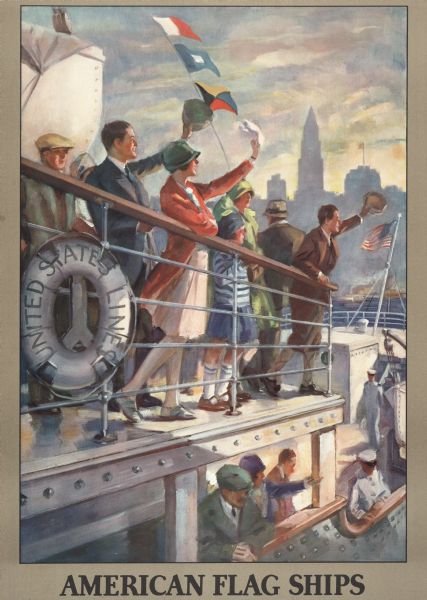The artwork depicts a bustling scene on an ocean liner, capturing a moment frozen in time. The image is reminiscent of a vintage print, roughly 8x10 inches, and framed by a thin light brown border that is slightly wider on the left and right, and noticeably broader at the bottom. Centered within this border, at the bottom, is a caption in bold, black, all-capital letters that reads "AMERICAN FLAGSHIPS."

Above the caption, an illustration, which resembles an oil painting but is actually a print, occupies most of the space. It features a group of people on the ship, standing by the railing. Some are cheerfully lifting their hats, waving—perhaps bidding farewell as the ship departs. They are dressed in a vintage style reminiscent of the 1940s, lending the scene an air of nostalgia.

Flying prominently at the front of the ship is an American flag, paralleled by three other flags at the top middle of the image—one white and red, and another dark blue and white. In the background, there are shadowy outlines or lights of buildings, suggesting a city skyline, likely New York City as inferred from the silhouette of what appears to be the Empire State Building. Above it all, the sky looms cloudy, adding a dramatic atmosphere to the scene.